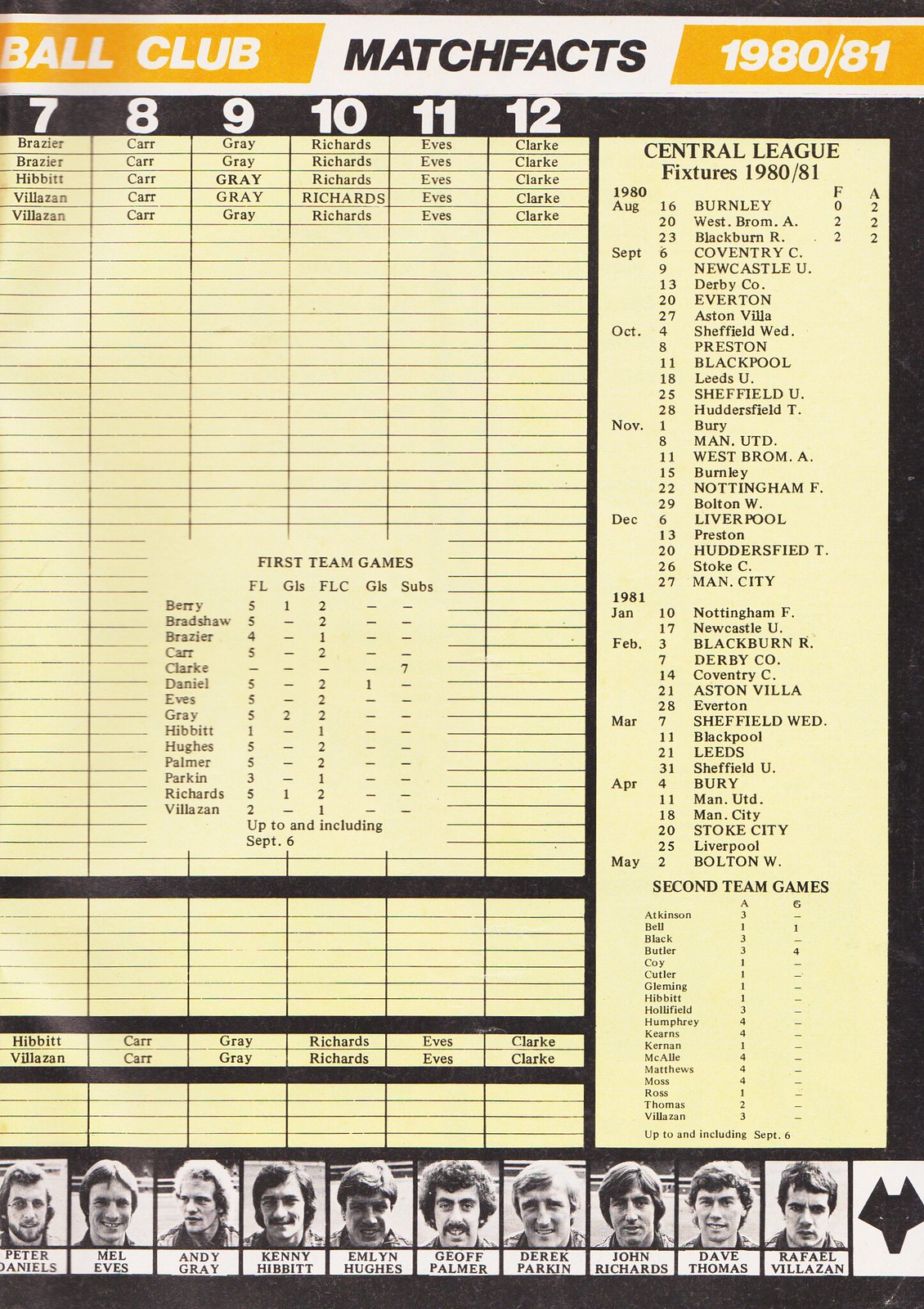The image features a detailed chart centered around "Central League Fixtures 1980/81." At the top, "Ball Club" is prominently displayed in white text on a yellow highlighted bar, followed by "Match Facts" in black text, and "1980/81" on another yellow highlighted bar. Along the black border at the top, numbers 7 through 12 are clearly visible. The main section holds a large, intricate chart featuring numerous tiny lines and letters.

To the right of the chart, there's a titled section "Central League Fixtures 1980/81," listing teams in small font, including Burnley, West Brom, and others. The list continues with mentions of Burnley, West Brom, Coventry C, Newcastle U, and many more, extending downwards. Below, there's a black line and additional text.

At the bottom of the image, there are black-and-white photographs of various men arranged in a row. Each man's face is accompanied by their name in black text on a white background. The names are Peter Daniels, Mel Evans, Andy Gray, Tony Hewitt, Emlyn Hughes, Jeff Palmer, Derrick Parkin, John Richards, Dave Thomas, and Raphael Bilazin. Adjacent to the last individual is a black clock head on a white background. Underneath the row of photographs is another black line, further contributing to the structured layout of the page.